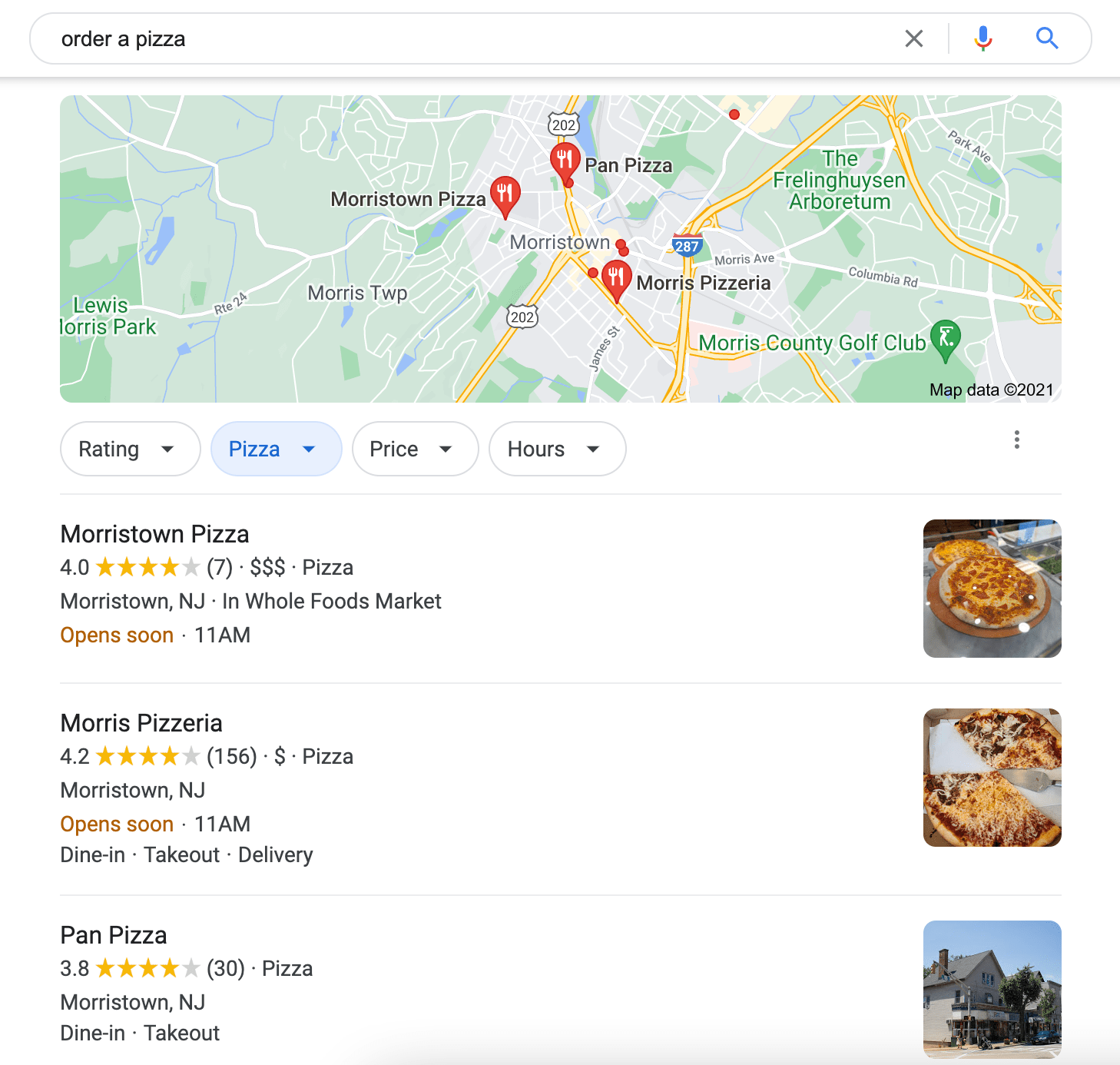This image is a screen capture from Google Maps on a tablet or smartphone, displaying search results for "order a pizza." At the top of the screen, an oval search bar with dark black text reads "order a pizza," flanked by a gray 'X' on the right, a microphone symbol, and a magnifying glass icon, indicating voice and text search options. 

Below the search bar, the map presents a street view populated with several red pins featuring white fork and knife icons, symbolizing restaurant locations. Just beneath the map, there are navigation tabs. The first circle, labeled "Rating" in black text, includes a down arrow. The second tab is selected, shown in blue text with a blue down arrow, indicating it is the active filter, with further options for "Price" and "Hours" visible alongside.

The first restaurant listed is "Morristown Pizza," rated at 4.0 stars based on 7 reviews. It features three dollar signs, denoting its price range, and labels itself as a pizza restaurant. Its location is noted as "Morristown, NJ," specifically inside "Whole Foods Market." The announcement "Open soon" is displayed in brown text, with an opening time of 11 a.m.

Following is another entry, "Morris Pizzeria," with a rating of 4.2 stars from 156 reviews, signified by a single dollar sign, indicating it is relatively inexpensive. Like the first, it is in Morristown, New Jersey. This establishment promises to open at 11 a.m., as highlighted in brown text. The listing also provides its service options: dine-in, takeout, and delivery.

The final restaurant shown is "Pan Pizza," carrying an overall rating of 3.8 stars from 30 reviews, though the visual suggests almost 4 out of 5 stars. It is labeled as a pizza place in Morristown, NJ, and offers only dine-in and takeout services.